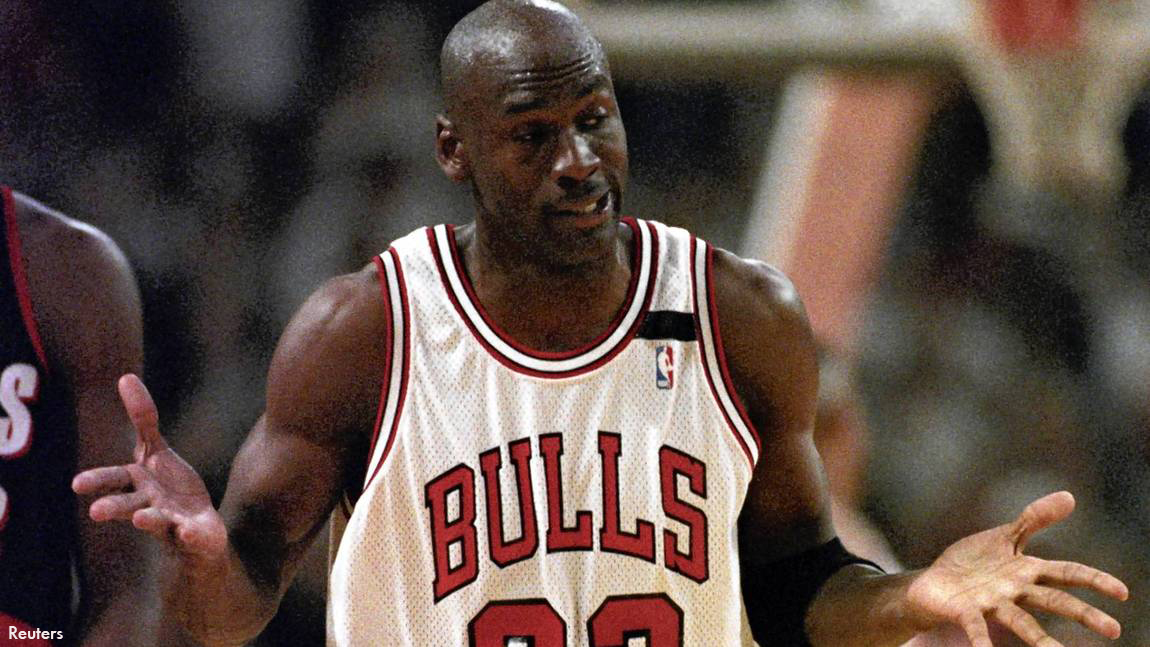This is a professional, full-color photograph of Michael Jordan during an away game, captured indoors with artificial lighting. The horizontally rectangular image focuses closely on Jordan, an African-American man with a bald head glistening with sweat under the lights, his black-brown skin contrasted by his white Chicago Bulls jersey adorned with red letters and the NBA logo on the left side. Although his jersey number 23 is partially obscured, you can discern the iconic design. Michael Jordan's expression is one of puzzlement, with his head slightly cocked and eyes looking to his left, both hands out in front of him, palms up, as if questioning a play. He also sports a black elbow pad on his left arm. In the out-of-focus background, the blue jersey of an opponent, likely from the Portland Trailblazers, is partially visible with only an 'S' discernible. The top right corner of the image shows a portion of the basketball net and backboard, while the bottom left corner features the white text "Reuters."